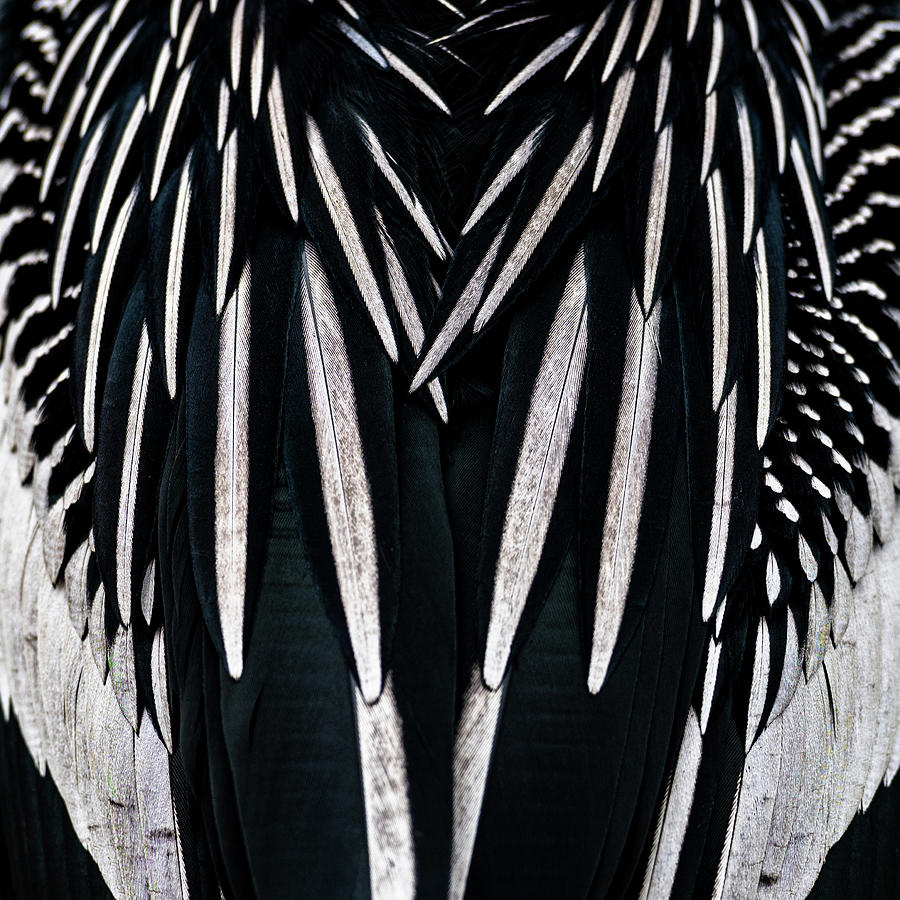This highly detailed black and white image features a striking close-up of an intricate array of feathers or feather-like structures. The photograph zooms in tightly, capturing just the back of what could possibly be a bird, angel wings, or an organic object resembling a seed pod. The image showcases an array of long, elongated oval feathers, each with a prominent white stripe down the center and black outlines on the edges. The feathers are densely packed, radiating symmetrically from the top of the image downwards, giving the appearance of a meticulously patterned, almost spiky texture. No other parts of the bird or object, such as the head, feet, or outer edges, are visible. The photograph's focus and extreme close-up perspective highlight the texturing and intricate details of the feathers, creating an almost surreal and abstract representation.